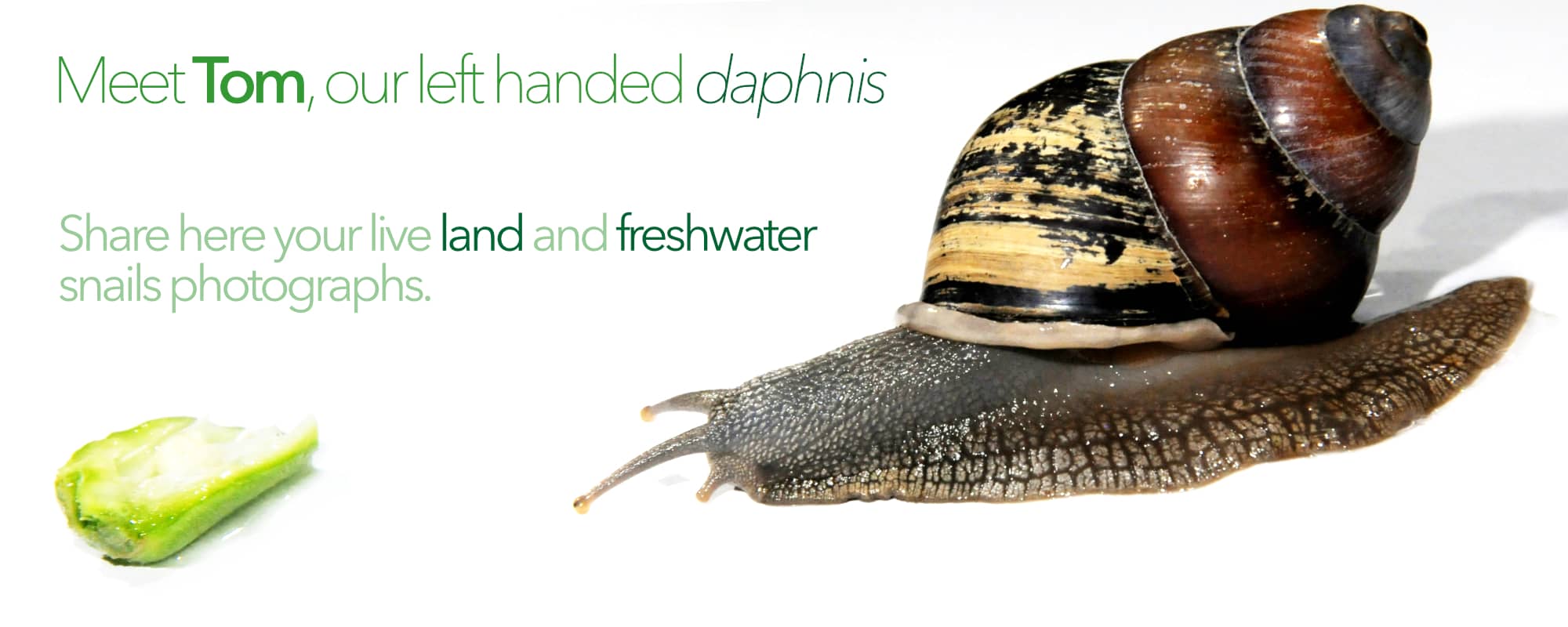The image depicts a detailed close-up of a large grayish-brown snail, with a strikingly colorful shell, crawling on a pristine white background. Positioned on the right side, the snail features a shell with gold and black bands at the forefront, transitioning into darker brown and gray spirals towards the back. The snail's body itself is a mix of gray, brown, and black, with visible eyes and antennae. To the left, close to the bottom of the frame, lies a piece of green vegetable, possibly a slice of celery or cut squash, towards which the snail is moving. Above the snail, in bold and italicized green text, the caption reads: "Meet Tom, our left-handed Daphnis." Followed by, "Share here your live land and freshwater snails photographs," with 'land' and 'photographs' in bold. A shadow is cast behind the snail, but the background remains completely white, highlighting the subjects.